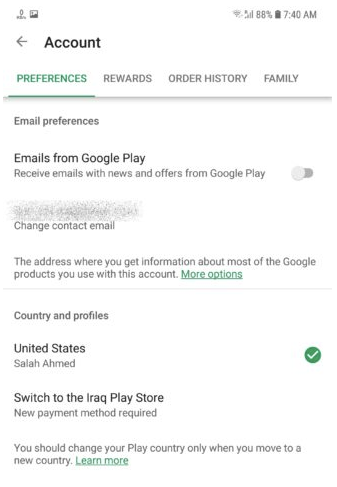**Screenshot of Google Account Settings on a Mobile Device**

At the top of the screenshot, the status bar on a white background displays various indicators: notification icons on the far left, and on the far right, the Wi-Fi signal icon, the cell tower signal strength indicator, and the battery icon showing 88% with the time "7:40 AM" to the right of it.

Below the status bar, a black arrow indicates a back button on the far left, leading to different settings. The navigation bar below this comprises options for "Preferences," "Rewards," "Order History," and "Family." The "Preferences" tab is highlighted in green, signifying it is currently selected.

Under the navigation bar, the screen displays:

- **Email Preferences:**
  - **Emails from Google Play:** A toggle switch for receiving emails from Google Play, which is currently turned off.
  - **Change Contact Email:** This section is blurred out to maintain privacy.

Below the email preferences section is a line of text indicating the address where one can receive information about most of the Google products used with the account, followed by a green link labeled "More options."

Further down, the screen details country-related settings:

- **Country and Profiles:**
  - **United States:** Displayed in bold with a green checkmark on the far right.
  - **Salah Ahmed:** This may indicate the user associated with the current account.
  - **Switch to the Iraq Play Store:** Displayed in bold, suggesting the option to switch the Play Store region.
  - **New Payment Method Required:** Indicating the need to update payment information to switch regions.

At the bottom of the screen, a cautionary note advises, "You should change your Play Country only when you move to a new country," accompanied by a green link labeled "Learn more."

The layout and structure of the settings page are organized to allow easy navigation and management of personal Google account preferences.